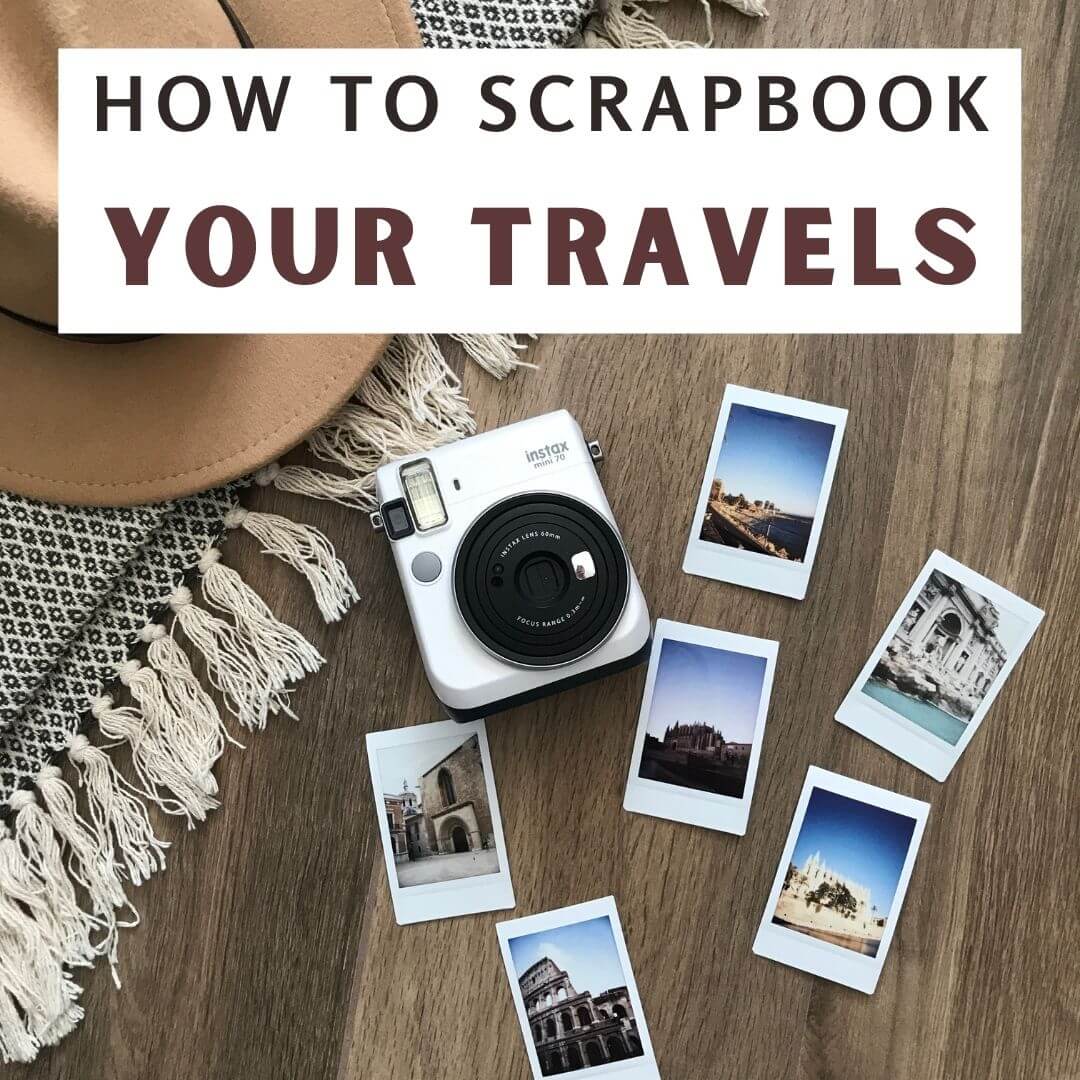The graphic, titled "How to Scrapbook Your Travels," features uppercase brown text for "YOUR TRAVELS" and white text for "how to scrapbook" within a white rectangle at the top. Below the title, a mocha brown cowboy hat with a ribbon rests on the top left corner, partially overlapping a hardwood floor backdrop. A black-and-cream diamond-patterned rug extends from the bottom left to the top middle, with intricate knots and frayed edges. Scattered on the wooden surface are six rectangular, white Polaroid-style photographs depicting various landmarks. A silver Instax camera, identifiable by its modern design, accompanies these photos. Each element—from the hat and rug to the pictures and camera—creates a visually rich guide to scrapbooking travel memories.